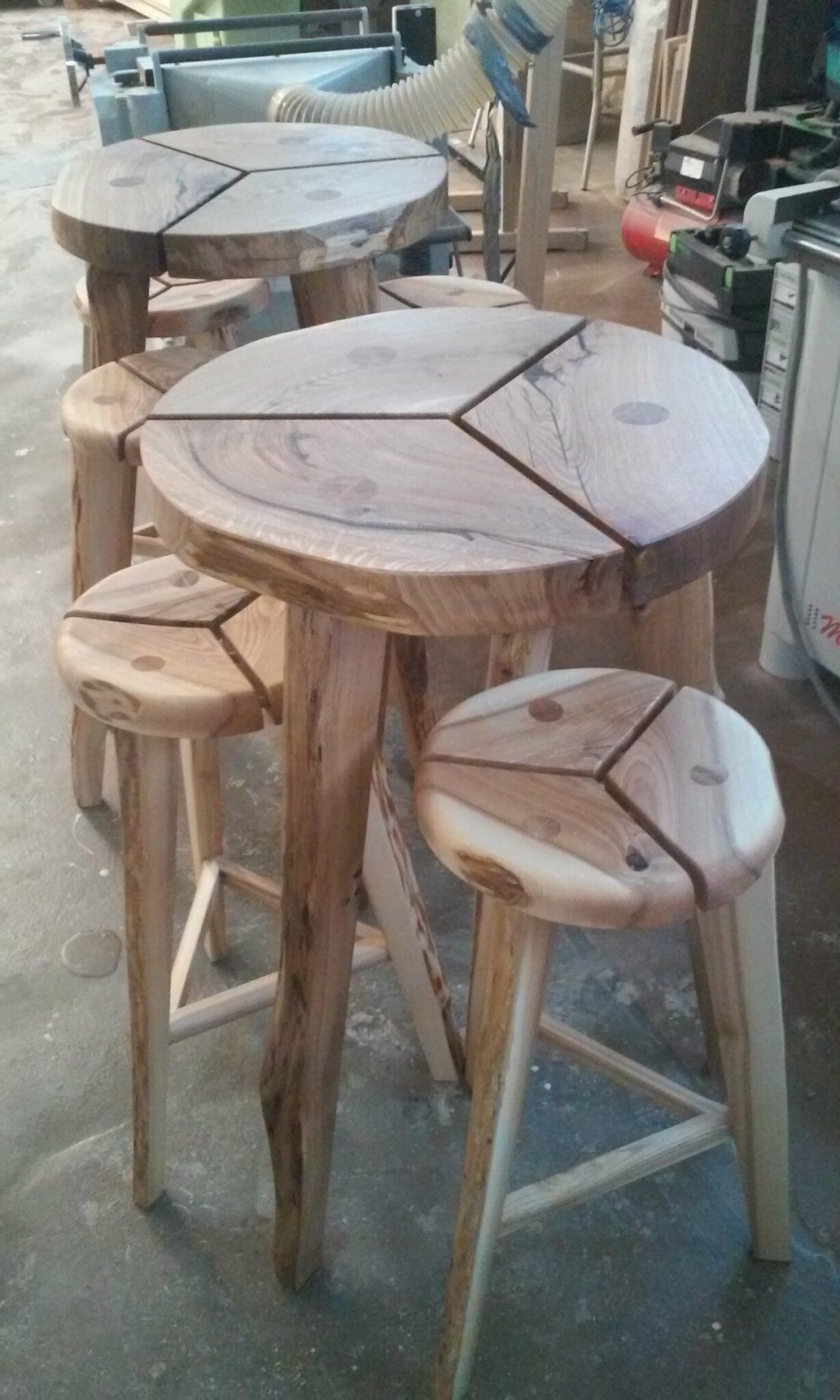The photograph depicts a rustic workshop environment within a warehouse-like setting, characterized by plywood walls and a variety of woodworking machinery. Prominent among the equipment is a large, gray machine accented with black bands, alongside a red machine with a black top and handle. Central to the image are two round wooden tables styled similarly, each split into a peace sign-like pattern, with three separate sections highlighted by visible lines. These tables, crafted from cross-sections of tree trunks, feature natural, reddish heartwood and light-colored sapwood, treated with a clear finish that preserves their raw aesthetic, including some bark along the live edges.

Accompanied by matching stools, the ensemble includes two sets of tables and stools, all exhibiting a consistent hand-crafted, rustic look. The stools have three angled legs with triangular bracing for stability, contrasting with the table legs, which are made from tapered branches or large limbs and lack such bracing.

Additionally, the image shows a large white tube taped at the joints, emerging from a metal vent and likely serving as an exhaust system for sawdust and debris. This tube connects to the woodworking machinery, underscoring the workshop setting. The arrangement of barstools and tables forms a diagonal line from the upper left to the lower right of the image, with some smaller stools slightly nested under larger ones, all polished to a smooth finish allowing the natural grain of the wood to stand out.